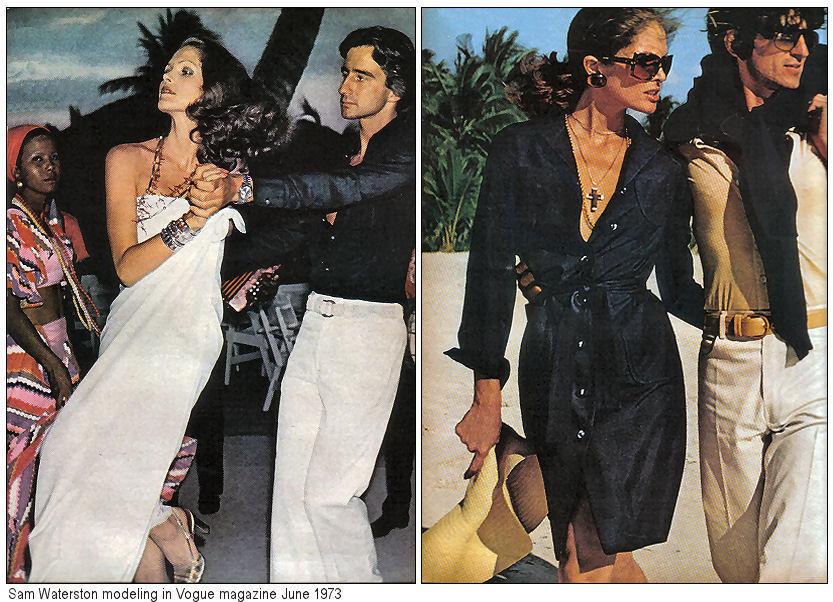The image depicts a split in a horizontal open magazine spread from Vogue, June 1973, showcasing two photographs of a young Sam Waterston, likely in his late 20s or early 30s. Each half captures a tropical setting with palm trees and a clear blue sky in the background.

In the left photograph, Sam Waterston is clad in a shiny black long-sleeve shirt paired with white trousers. He is seen dancing with a beautiful woman who has long, dark hair and is dressed in a strapless white gown adorned with heavy necklaces. They are holding hands, with Waterston's left arm extended and the woman's right arm bent, clasping his hand. Behind them, white chairs and tables are visible along with another woman dressed in a vibrant pink, red, and green printed top and skirt, accessorized with a red headscarf, metallic earrings, and a long necklace. This woman appears to be of African descent.

The right photograph also features Sam Waterston, who now sports sunglasses, a tan shirt, light tan khakis, and a black scarf draped around his shoulders. He is walking on a beach with a large grove of palm trees in the background. Arm in arm with him is the same dark-haired woman, now wearing a black, low-cut button-down dress belted at the waist. She holds a straw sun hat in her right hand. Both appear to be looking to their right, immersed in the picturesque tropical surroundings.